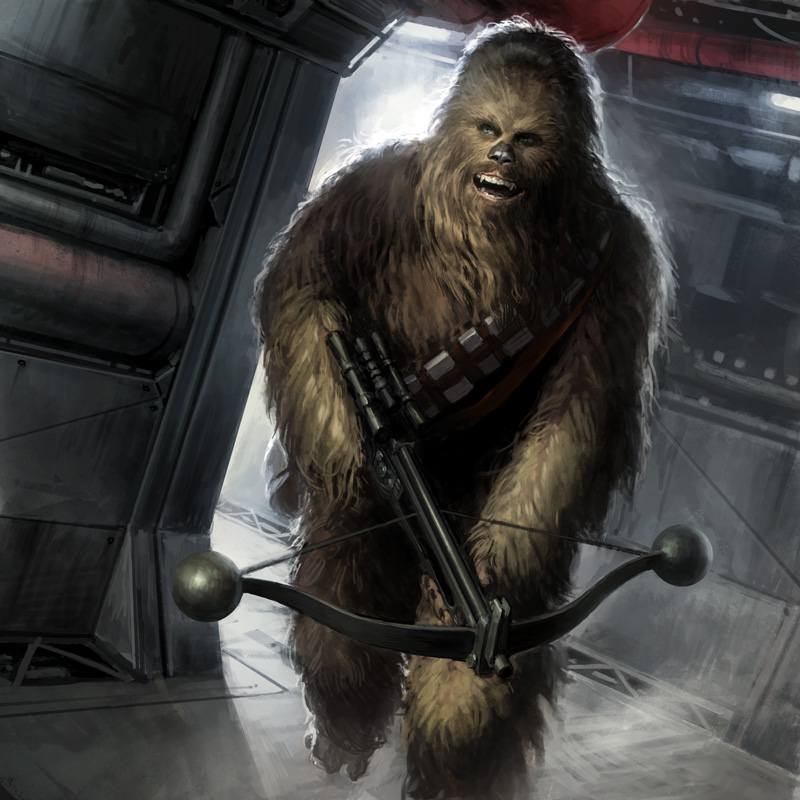In this vividly detailed animated image inspired by Star Wars, we see Chewbacca charging through the corridor of a futuristic spaceship. The hallway's color scheme is primarily gunmetal gray, with industrial walls and floors, adding to the authentic sci-fi atmosphere. Chewbacca, depicted front and center, is holding a black crossbow, cocked and ready to fire, with two spheres on either end. His iconic ammo belt is slung from his left shoulder to his right hip. Chewbacca's mouth is open, revealing his white teeth and prominent fangs, as he appears to be running directly toward the viewer. His brown fur showcases various shades, adding depth to his character design. A beam of light silhouettes his figure from behind, illuminating a doorway. Additional red accents appear on the left and in the top right corner of the image, highlighting parts of the spaceship. A red pipe at the top right corner adds a touch of color contrast to the otherwise monochromatic setting.